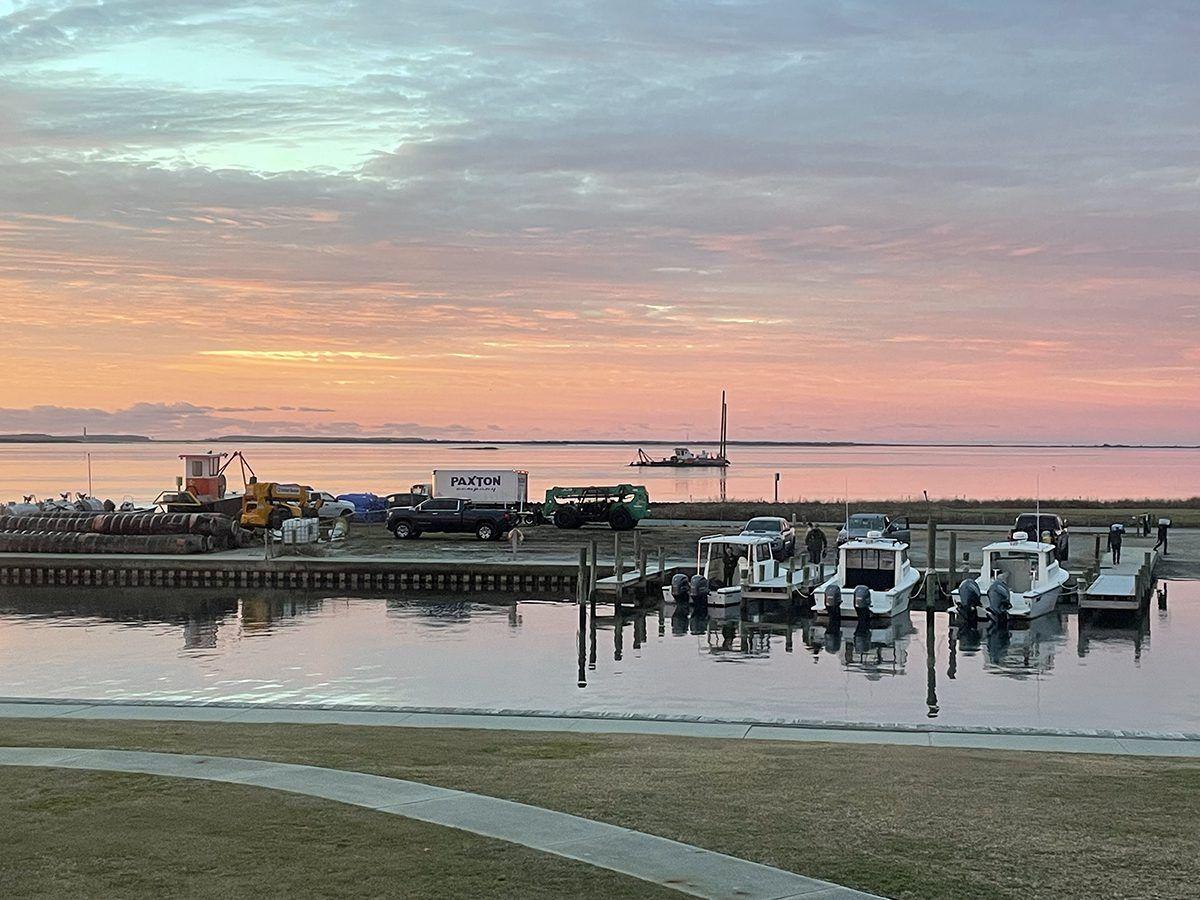The photograph depicts a serene marina scene with an unfinished dock jutting out towards an expansive sea, where the sky meets the water at a distant horizon painted in pale hues of blue, grey, pink, orange, and gold. In the foreground, a sandy area features a paved footpath leading to the water's edge, where several yachts and motorboats are moored next to small docks supported by pylons. On the left side, black rolled-up tarps or fabric are visible, while pallets with goods ready for loading dot the docks. Across a narrow strip of water lies another strip of land with a road running through it, lined with an assortment of vehicles including a blue pickup truck, a white container truck labeled "Paxton," a trailer, and several other cars. A person stands by, observing the tranquil scene, while a small boat glides across the water in the background. The overall image captures a busy yet peaceful marina bathed in soft, pastel colors.